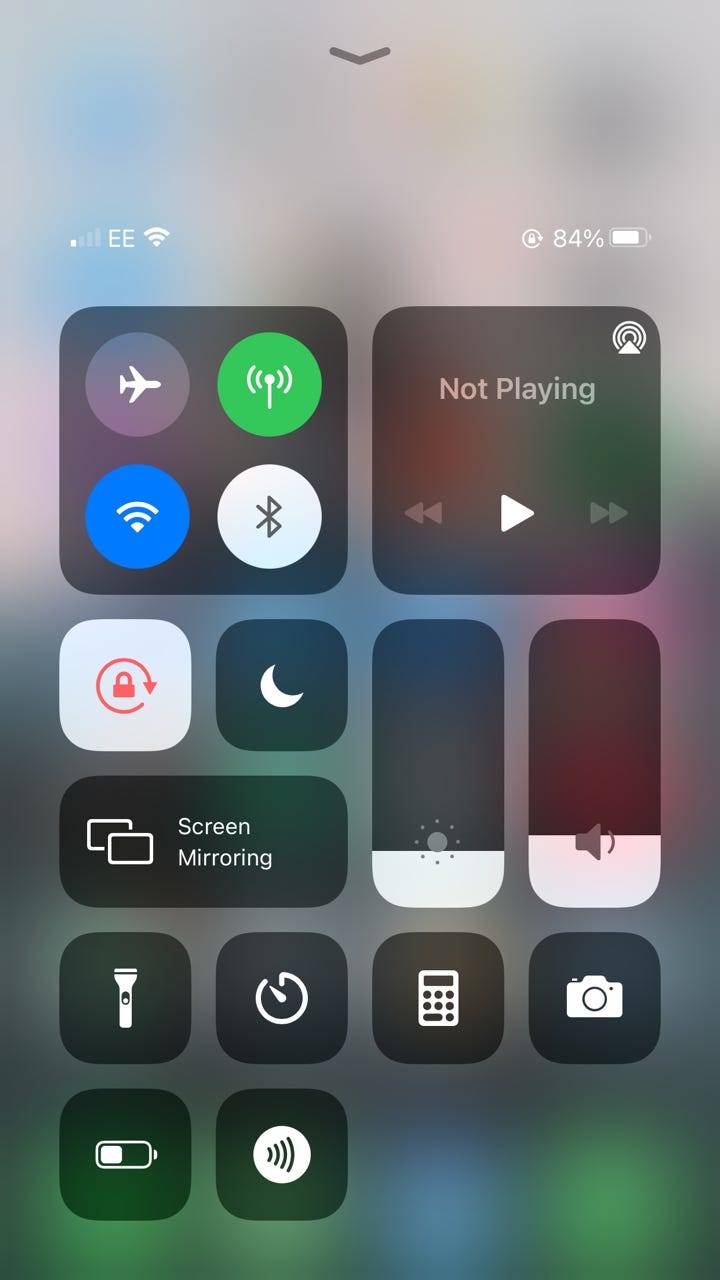This image captures the control center page of a smartphone. At the top, a small gray downward-facing arrow is prominently featured. Below this, indicators for both Wi-Fi and cellular network connectivity are visible, with the cellular signal showing only one bar and labeled with the letters "EE." To the right of these indicators, a rotation lock symbol and a battery percentage reading of 84% are displayed.

Further down, a row of functional buttons is neatly aligned, including an airplane mode icon, a Wi-Fi indicator with a blue background, a cellular signal icon with a green background adorned with a cell tower symbol, and a Bluetooth icon on a white background. Additionally, a red-lit rotation lock icon is shown, indicating it is currently active.

A "Now Playing" box occupies the center, complete with navigation arrows for back, play, and forward functions, facilitating media control. Adjacent to this are icons for various utilities such as a crescent moon symbol for Do Not Disturb mode, brightness and volume sliders filled to about one-third with silver color, a screen mirroring button, a flashlight toggle, a stopwatch, a calculator, a camera icon, a battery icon, and a sound customization button denoted by a series of lines.

Together, these elements provide a comprehensive interface for managing device functions and settings.